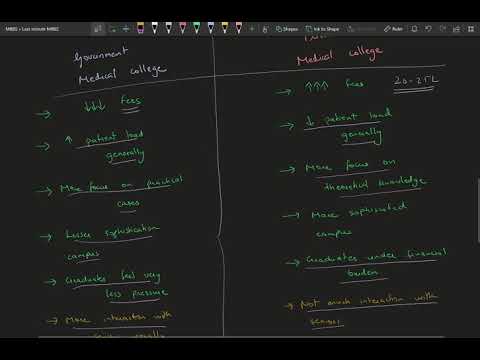The image depicts a screenshot from a computer screen running a software program that appears to be used for drawing or editing. The entire screen has a predominantly black background, resembling a digital blackboard. At the top of the screen, there is a menu bar with various tiny, unreadable options and tools, including icons representing a marker, eraser, and color selections shaped like pencil tips in hues such as pink, white, gray, red, green, yellow, and orange. 

The main section of the screen is divided into two halves with handwritten text that is difficult to read, suggesting that it was written using a touch screen or a stylus. The left side of the screen features a list that possibly reads "Government Medical College," written in white with green arrows pointing to six different entries. The right side also has a heading related to a medical college with text and arrows, five of which are in green and the remaining two are in yellow, though the details remain blurry due to the low resolution of the image. This setup indicates a comparison of some kind, possibly listing positives and negatives or different attributes, as suggested by the structure and use of arrows. The overall appearance is reminiscent of a simulated blackboard used in an educational context, likely for a college course.